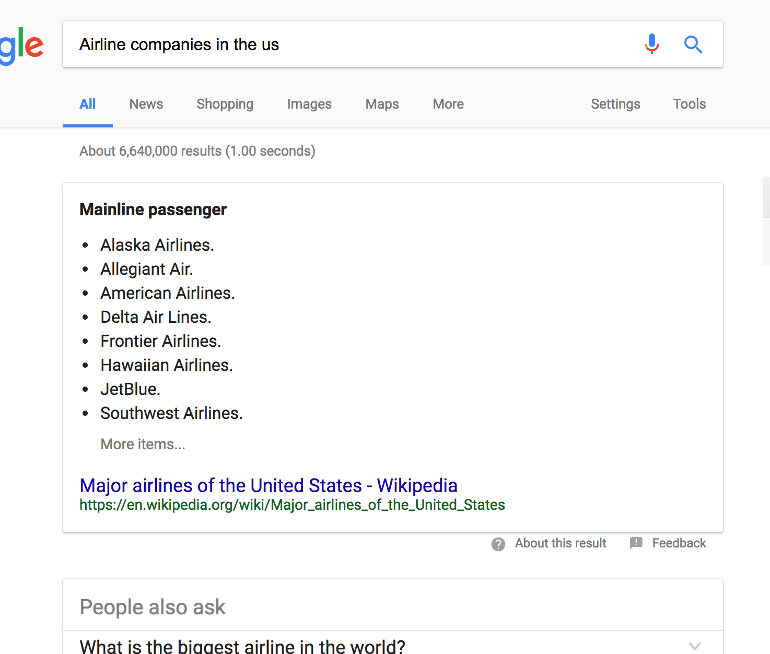The image captures a partial web page from Google. In the upper left-hand corner, the tail end of the Google logo is visible, specifically the letters "GLE." The main feature is the Google search bar, which contains the query "airline companies in the U.S." Displayed below the search bar, there's an indication of about 6,640,000 search results. The top result visible is a snippet from a Wikipedia page, listing eight mainline passenger airline companies in the United States. These airlines are presented in a vertical, bulleted list: Alaska Airlines, Allegiant, American, Delta, Frontier, Hawaiian, JetBlue, and Southwest. The search result also includes a link to the corresponding Wikipedia page titled "Major airlines in the United States - Wikipedia." The background of the image is predominantly white, featuring a light gray banner at the top for additional visual structure.